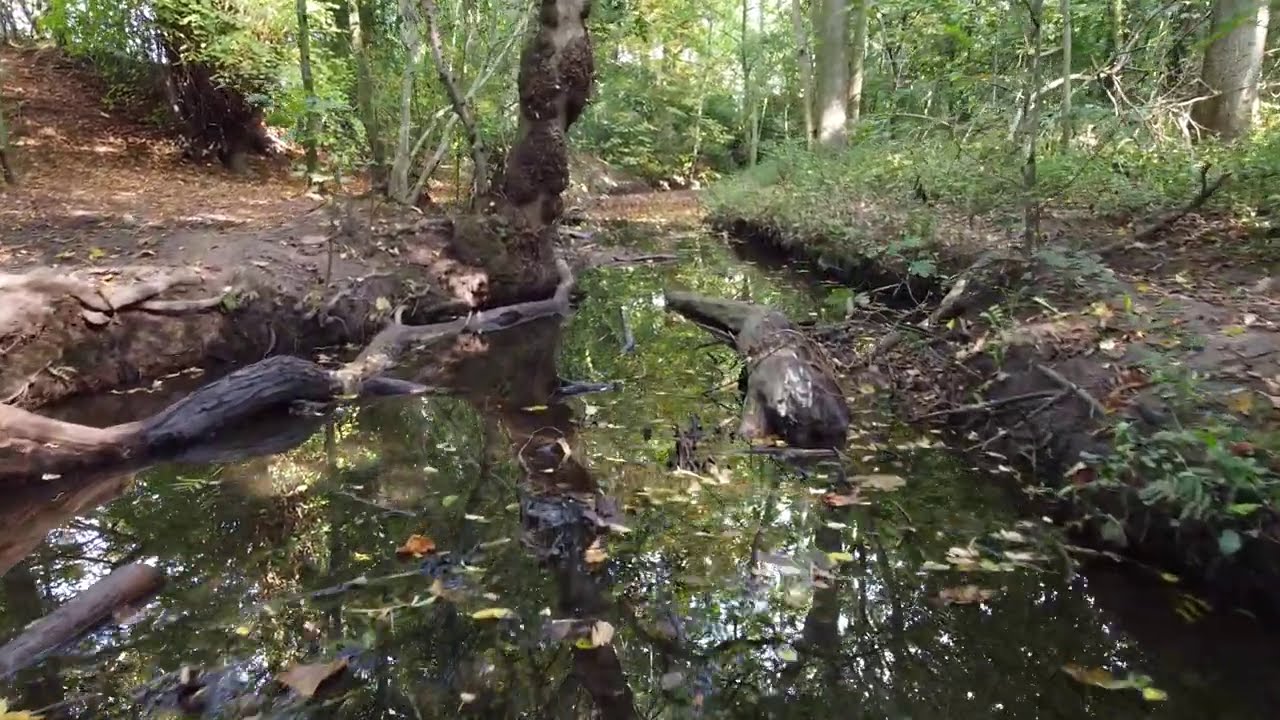This photograph captures a serene but wild wetland scene in the heart of a forest. Central to the image is a small creek or stream, its murky, dark water scattered with floating leaves and fallen branches, emanating an untamed, natural charm. To the left of the stream lies a patch of bare, dark brown earth dotted with sticks, leaves, and the roots of young trees and shrubs. The right side of the image features a mix of dense greenery and brush, possibly hiding something shiny and wet, such as a piece of wood coated in slime or even an elusive alligator, partially submerged and blending into the environment. The vivid array of colors, including shades of brown, green, tan, white, and clear water, are accentuated by sunlight filtering through the canopy above. The backdrop is framed by a variety of tree trunks, both thick and slender, creating a dappled pattern of light and shadow. Overall, this outdoor snapshot encapsulates the raw beauty and diversity of a woodland wetland, embodying the tranquil yet dynamic ecosystem.